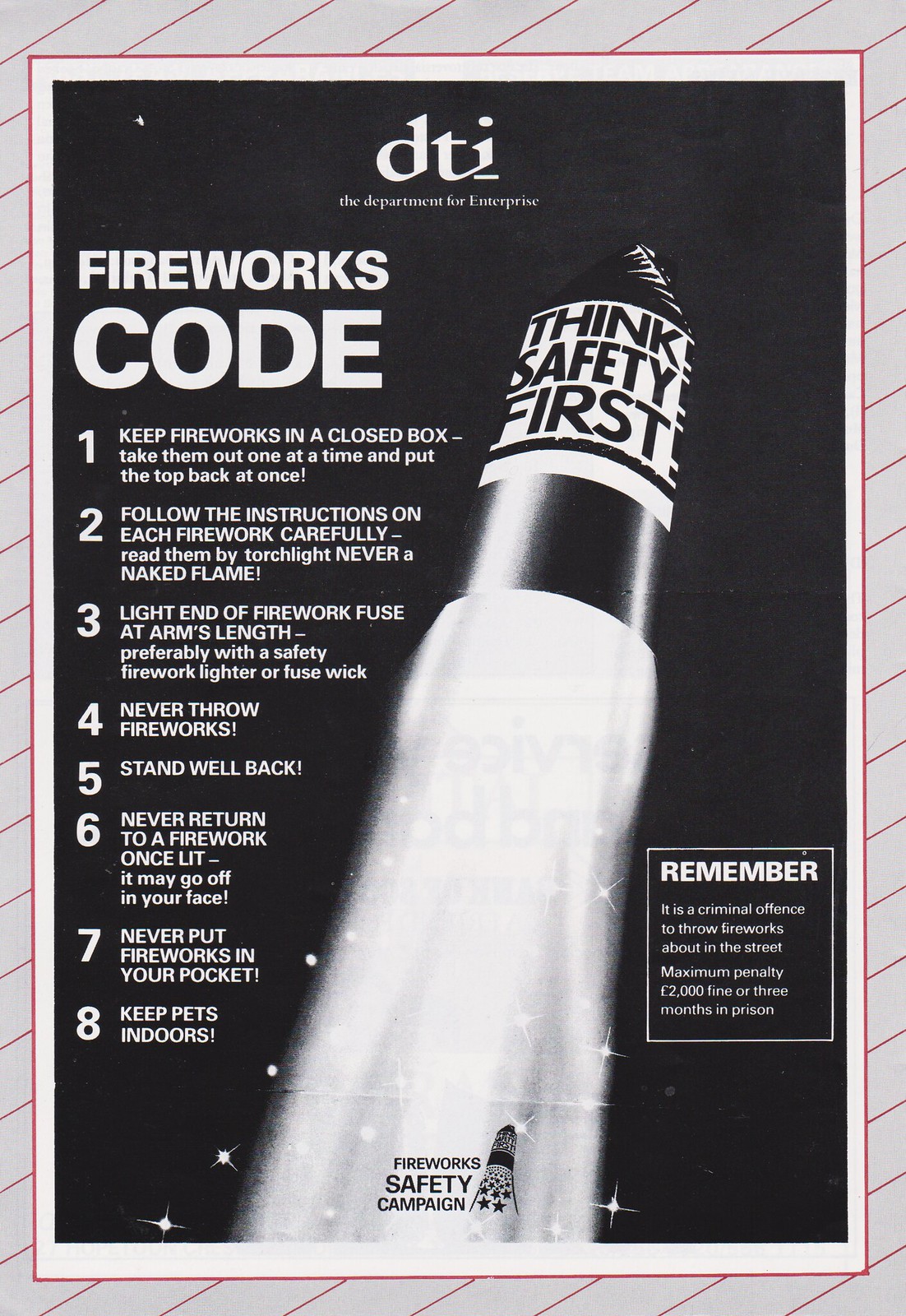This image is a flyer focused on fireworks safety, designed by the DTI, the Department for Enterprise. The flyer has a prominent black background with white lettering. Central to the design is an image of a vibrant rocket, generating flames and sparkles, labeled with a banner that reads, "Think Safety First." At the top of the flyer, in bold letters, it states "DTI, the Department for Enterprise," while at the bottom, it says "Fireworks Safety Campaign." 

On the left side of the flyer, the "Fireworks Code" is outlined in large white letters, detailing eight crucial safety rules:
1. Keep fireworks in a closed box. Take them out one at a time and put the top back at once.
2. Follow the instruction on each firework carefully. Read them by torchlight, never a naked flame.
3. Light the end of the firework fuse at arm's length, preferably with a safety firework lighter or fuse wick.
4. Never throw fireworks.
5. Stand well back.
6. Never return to a firework once lit. It may go off in your face.
7. Never put fireworks in your pocket.
8. Keep pets indoors.

To the right, in a white-bordered square, a strong warning in large white letters says, "Remember, it is a criminal offense to throw fireworks about in the street. Maximum penalty, £2,000 fine or three months in prison." The flyer is completed with a red-striped gray border, emphasizing the importance of safety during fireworks use.